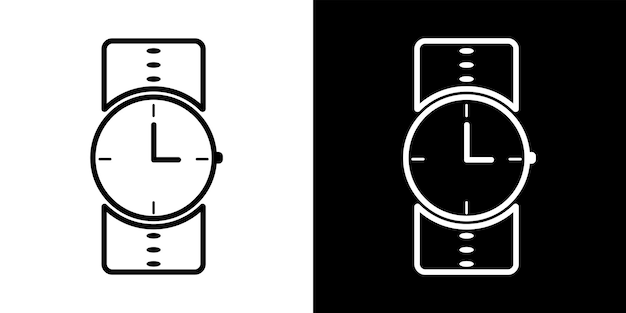This image showcases two starkly contrasting, digitally rendered depictions of a wristwatch. On the left, against a pristine white background, the watch is outlined in bold black. The round watch face is minimalist, featuring only four dashes at the 12, 3, 6, and 9 o'clock positions. It's set precisely to 3 o'clock, with two black hands indicating the hours and minutes. An outlined knob for winding protrudes from the right side, and the bands above and below the face extend outward, each displaying three small notches that suggest adjustable strap holes. On the right, the second image presents an inverse version; a striking black background envelops a watch outlined in crisp white. The hands again indicate 3 o'clock, preserving the symmetry between the two images. Every detail is mirrored, from the winding knob to the strap notches, emphasizing the stark contrast in color scheme while maintaining identical design elements.